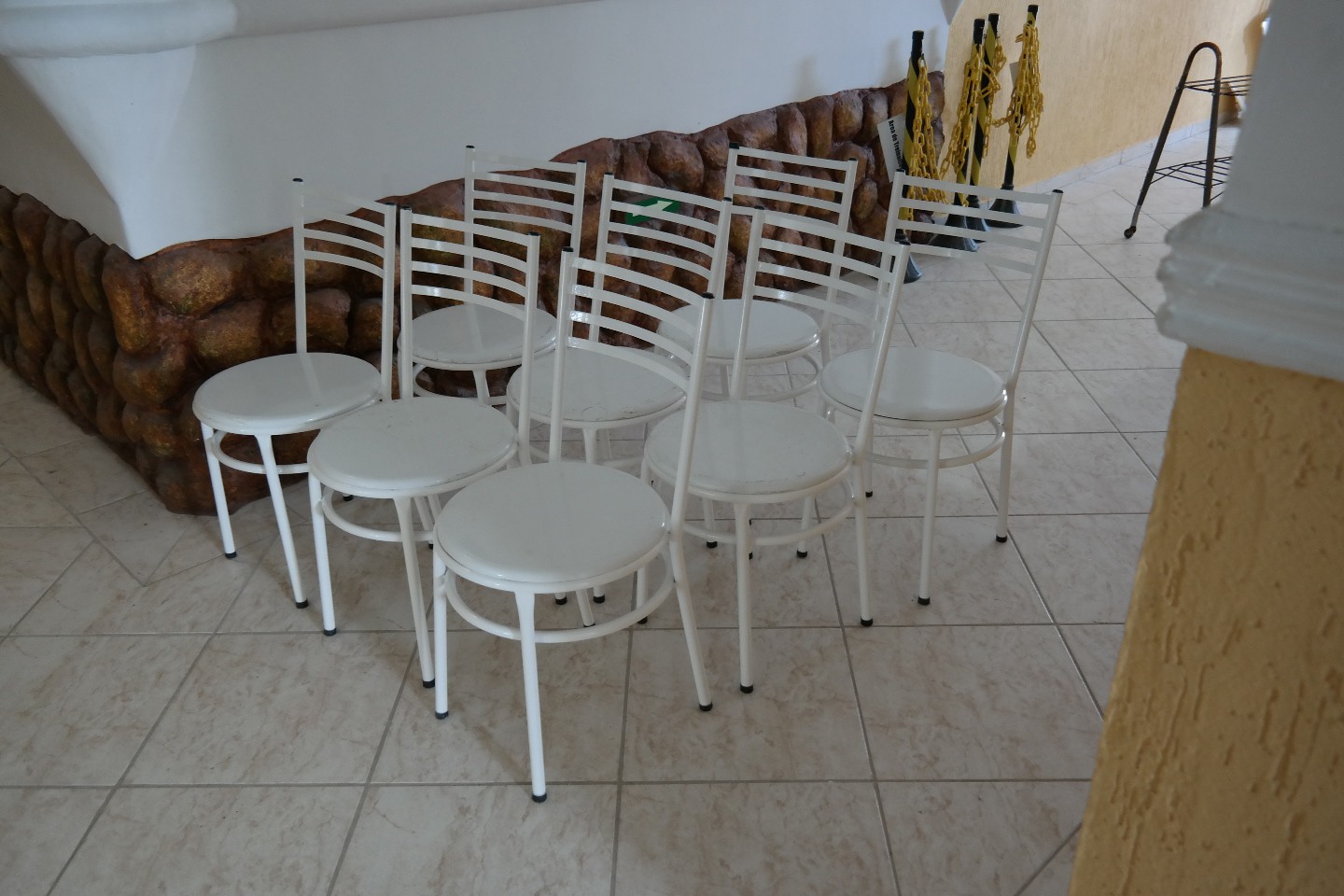The image depicts an indoor setting with eight white metal stool chairs lined up in a pattern across three rows: three chairs in the first row, three in the second row, and two in the third row. Each chair features a white steel frame with a round steel seat and a lower ring connecting the four legs, just beneath the seat. The floor underneath is tiled with light brown markings, and in the background, there is a steel structure and a large object covered with a white sheet. The room also includes a light-colored wooden door, part of a wooden floor, and a two-shelf metal unit visible to one side. The precise architectural style hints at a formal or possibly European setting, suggesting the possibility of a ceremonial or formal environment.